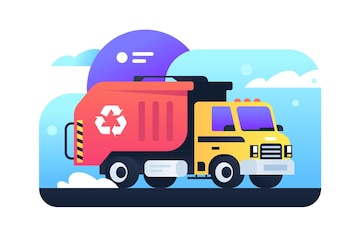This is a small, cartoonish digital illustration that looks like clipart, possibly an icon for an app. It features a recycling truck with a yellow cab and dark blue, almost purple-tinted windows. The truck has a silver bumper and is shown on top of a thin black line representing the road. The back of the truck is red with a white recycling symbol on it, indicating its use for recycling. It appears to be moving fast, as suggested by the white cloud of dust near the back wheel. The background depicts a light blue sky with a few stylized white clouds. Above the truck, there is a prominent dark purple crescent shape, giving the impression of a crescent moon.